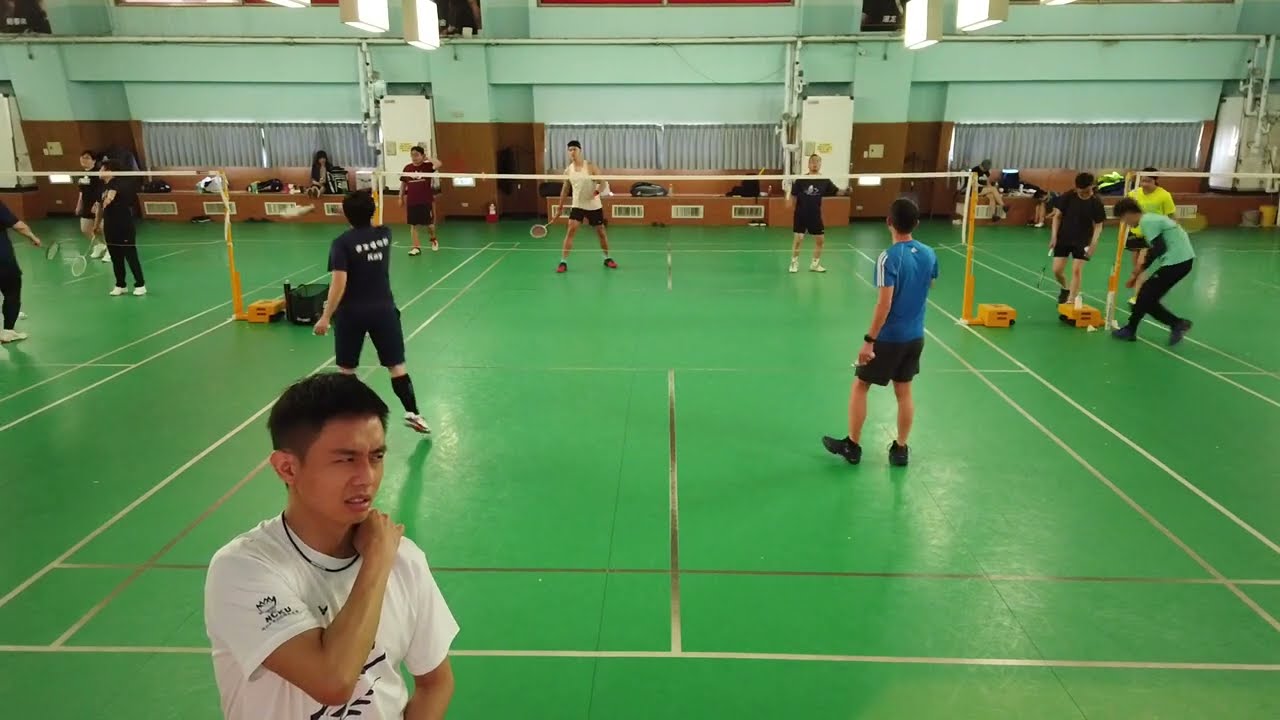This color photograph captures an indoor badminton facility with a bright, well-lit setting. The image features three adjacent badminton courts, distinguished by their green floors and white lines, separated by yellow-pole nets. On the central court, a man in a white t-shirt stands with a confused expression, his arm resting over his shoulder. Nearby, four players are actively engaged in a game. To the right, three individuals are walking towards the center of their court, with two bending down, possibly to retrieve a shuttlecock. On the left court, players appear to be pausing between plays. Surrounding the scene, the walls are painted a pistachio color, adorned with brown doors, wall panels, and gray windows with closed shades. The gym's numerous participants, primarily dressed in shorts or black pants, animate the bustling space.